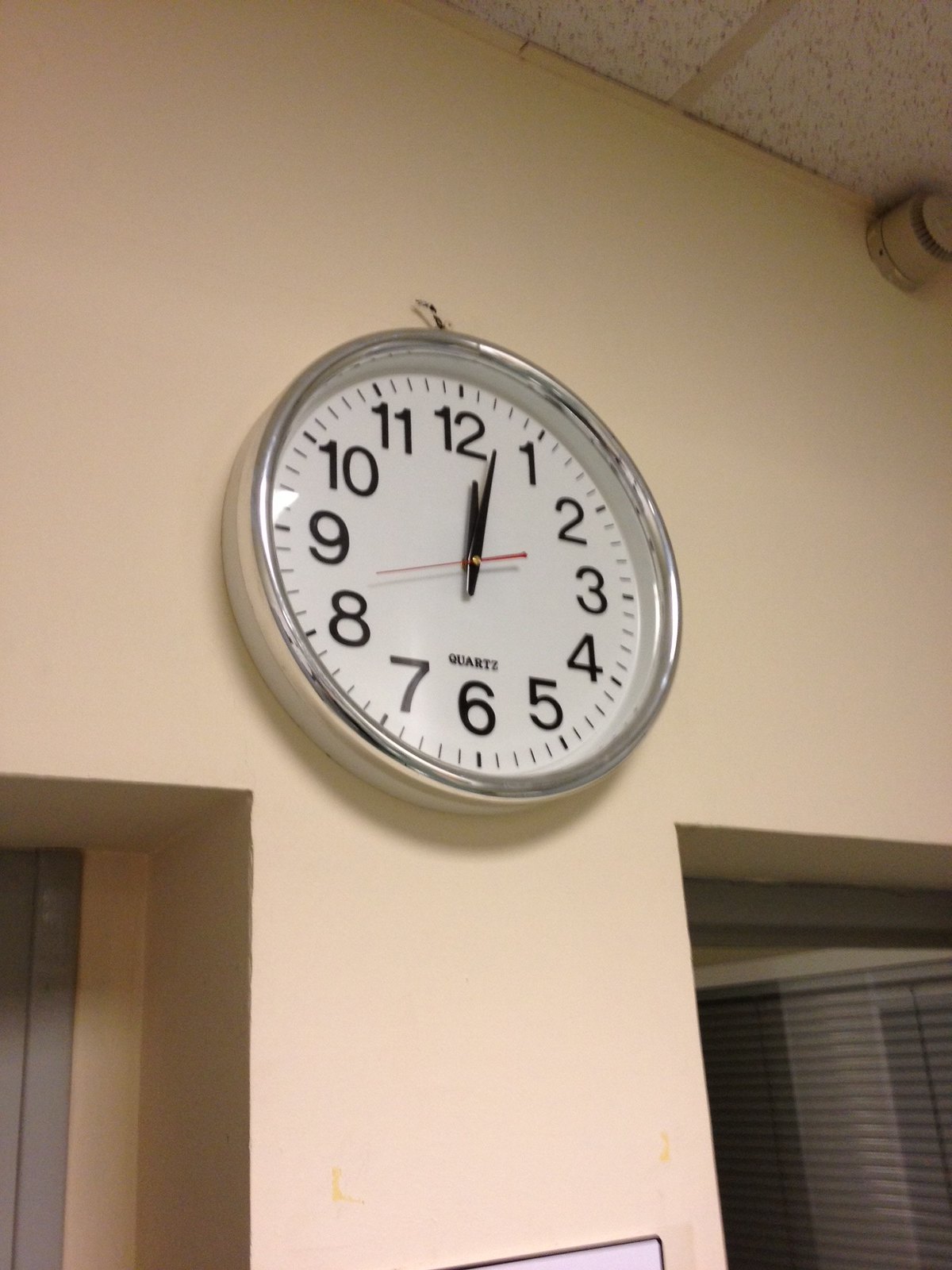This photograph appears to be taken inside a building, perhaps a house, classroom, or office, characterized by a peach-colored wall that dominates the image. High on the wall, slightly right of center, is a silver-framed clock with a white face, black block numbers, and thin black hands indicating the time is just past twelve o'clock, along with a red second hand pointing between the 8 and 9. The word "Quartz" is visible on the clock face. At the top right corner of the image, part of what seems to be a white-tiled ceiling is visible, accompanied by a smoke or fire alarm below it. The wall separates into what looks like a T-section, adorned with peach-colored lines that match the wall. To the left and right edges at the bottom of the wall are two doorway-like openings. The left side reveals a gray area that might be a wooden door frame, while the right side shows a window with white blinds or possibly a curtain, accentuated with light gray and darker stripes.